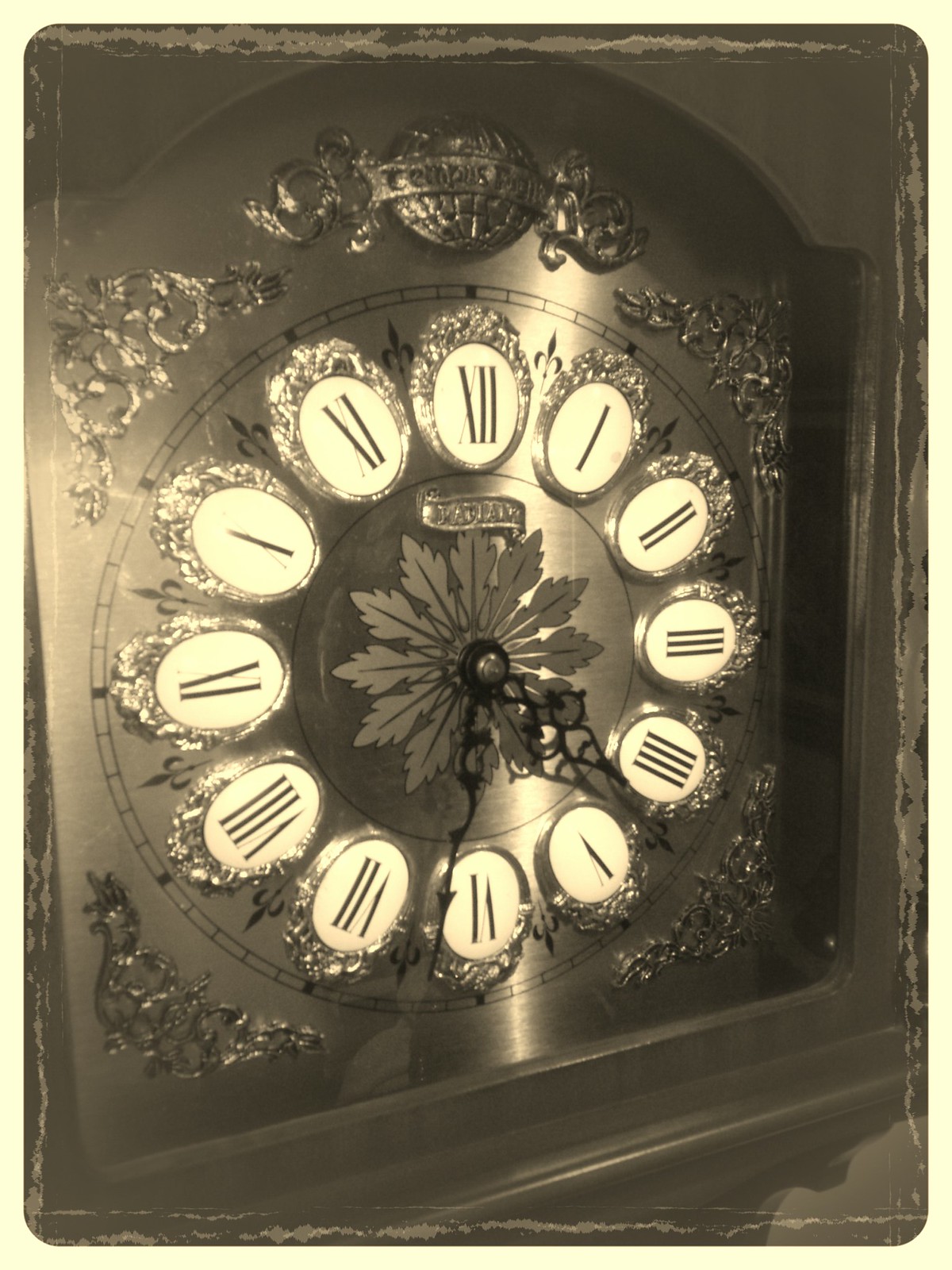This photograph showcases a highly ornate and old-fashioned clock, rendered in a sepia tone, which gives it a vintage appearance. The clock is square in shape with a face likely made of a metallic material such as gold or brass. Both Roman numerals and detailed embellishments decorate its surface. Each numeral from I to XII is mounted on a white, possibly ceramic, background and encased in a decorative metal frame. The center of the clock face features a flower or leaf-shaped design from which the clock hands extend. The minute hand is positioned just after the VI, while the hour hand is between III and IV, indicating that the time is approximately 3:31 or 3:32. The clock is also adorned with intricate leaf and scroll designs on its corners, and a round object, possibly a globe or crest, sits atop the clock. This ornate piece appears to be mounted on a wall, which could be white or gray, and features a small shelf below it.